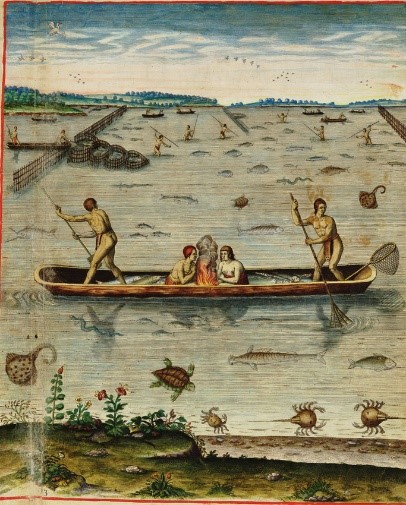This artwork, either a painting or a detailed drawing, portrays an ancient fishing scene with longboats under a blue, partly cloudy sky. The horizon is marked by a tree-lined shoreline, emphasizing a natural setting. In the foreground, fishermen wearing loincloths are depicted in the longboats, with two individuals seated in one boat and two others standing at either end holding oars. Alongside them, intricate nets are drawn, and varied sea creatures like turtles, bass, northern pikes, gars, starfish, jellyfish, and crabs are vividly illustrated as if seen beneath the water's surface. Further back, more boats are visible with people working using spears, similarly dressed in loincloths, and various fish traps are scattered throughout the scene. The imagery combines elements both above and below the water, creating a layered depiction of ancient aquatic life and fishing practices.